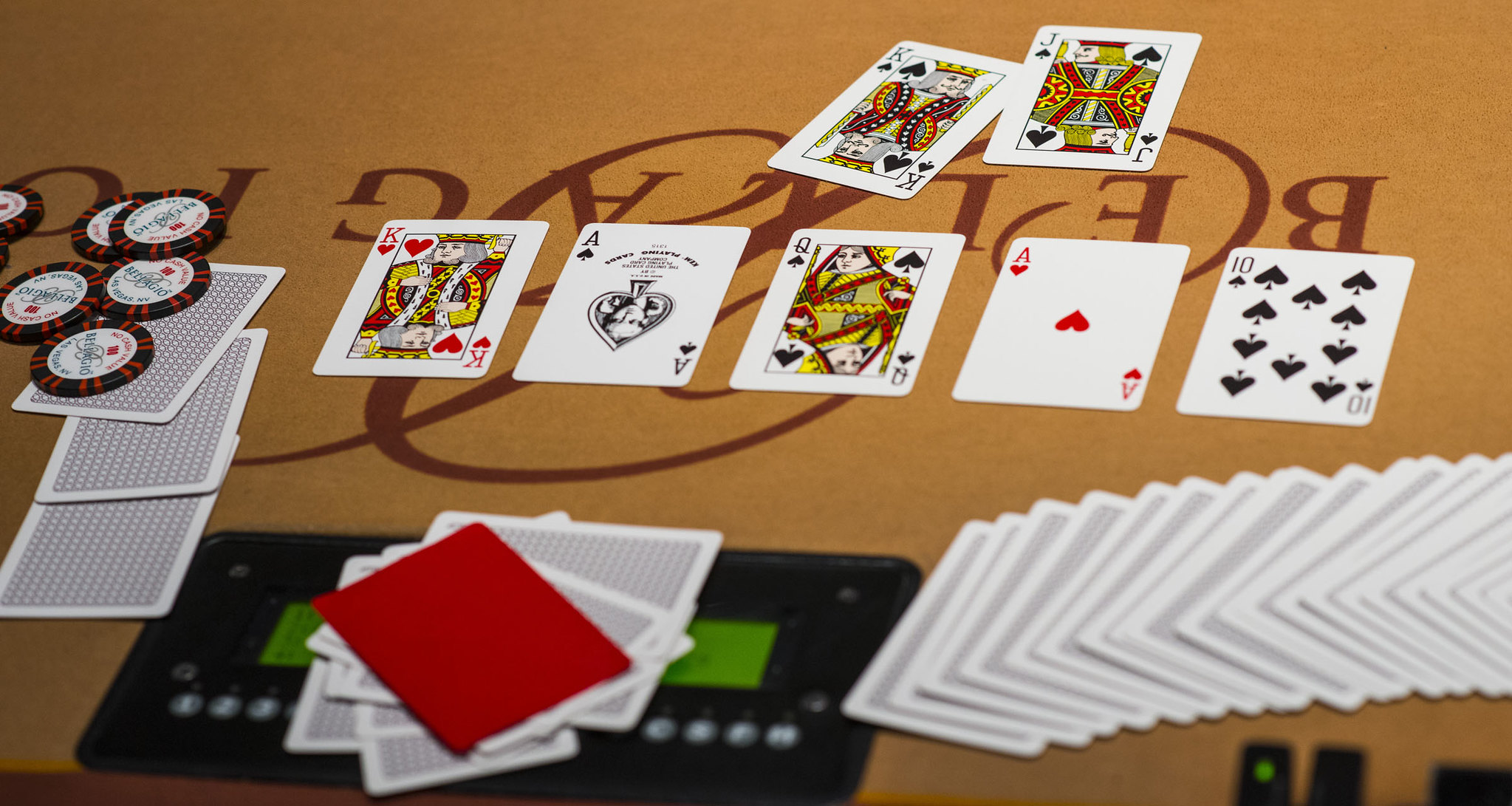The photograph captures a close-up view of a poker table adorned with a beige felt surface featuring the "Bellagio" logo in darker brown text, albeit upside down. Scattered across the table are a deck of playing cards, mostly lying face down, with around seven cards prominently face up displaying a variety of ranks and suits including the King, Queen, Ace of Spades, Ten of Spades, and Ace of Hearts. On the left side, there is a small stack of poker chips. A single red card stands out in the lower portion of the image. Adding to the scene, several partially visible electronic devices are embedded into the table, each featuring buttons labeled with numbers and various symbols, along with a green display situated beneath some of the cards.